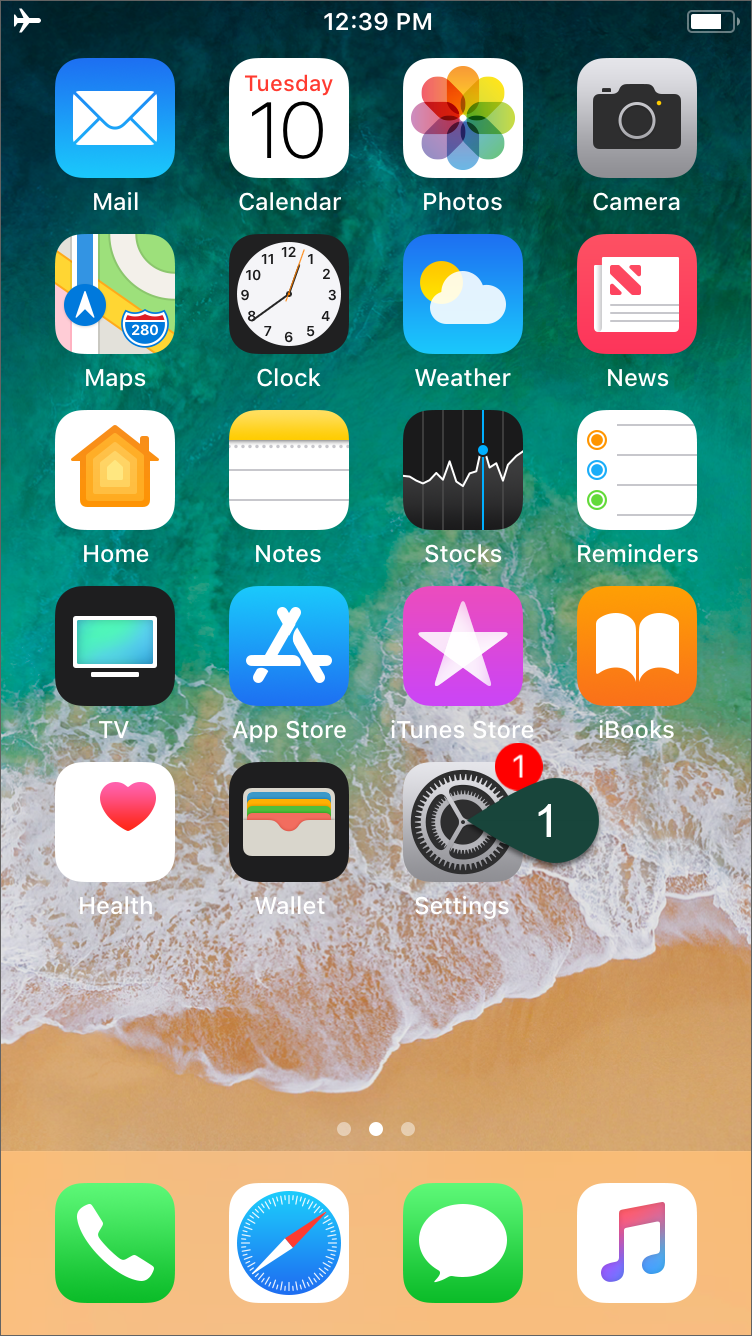This image displays a screenshot of an iPhone home screen captured at 12:39 PM. The device is in Airplane Mode, and the battery level is approximately 75% charged. The background image features a serene beach scene with a wave gently coming up onto the shore.

The screen is populated with various app icons, each meticulously identifiable. From top to bottom and left to right, the icons are:

1. Mail: A blue square with a white envelope.
2. Calendar: A white square indicating "Tuesday the 10th."
3. Photos: A rainbow-colored, flowery pinwheel.
4. Camera: A gray square with a black camera icon.
5. Maps: Illustrated by a map icon.
6. Clock: A standard clock face.
7. Weather: A blue icon with a cloud and a sun.
8. News: A red icon showing a piece of paper with an 'N.'
9. Home: A yellow house in a white square.
10. Notes: A white square symbolizing a piece of notebook paper.
11. Stocks: A white line graph on a black background.
12. Reminders: A white piece of paper icon with buttons colored orange, blue, and green.
13. TV: A black square displaying a TV monitor.
14. App Store: A blue icon with a white 'A.'
15. iTunes Store: A purplish square with a white star.
16. iBooks: An orange square featuring a white book.
17. Health: A white square with a red heart.
18. Wallet: A black square resembling cards in a wallet.
19. Settings: A gray cogwheel with a red notification badge marked '1.'

At the bottom of the screen are the user’s frequently used apps:

1. Phone: A green square with a white phone icon.
2. Safari: A white square with a blue compass.
3. Messages: A green square with a white speech bubble.
4. Music: A white square with a multicolored music note.

Additionally, a small teardrop-shaped indicator appears on its side, also marked with '1,' suggesting a pointed notification. Thin dots are visible at the bottom, hinting at the presence of additional home screens.